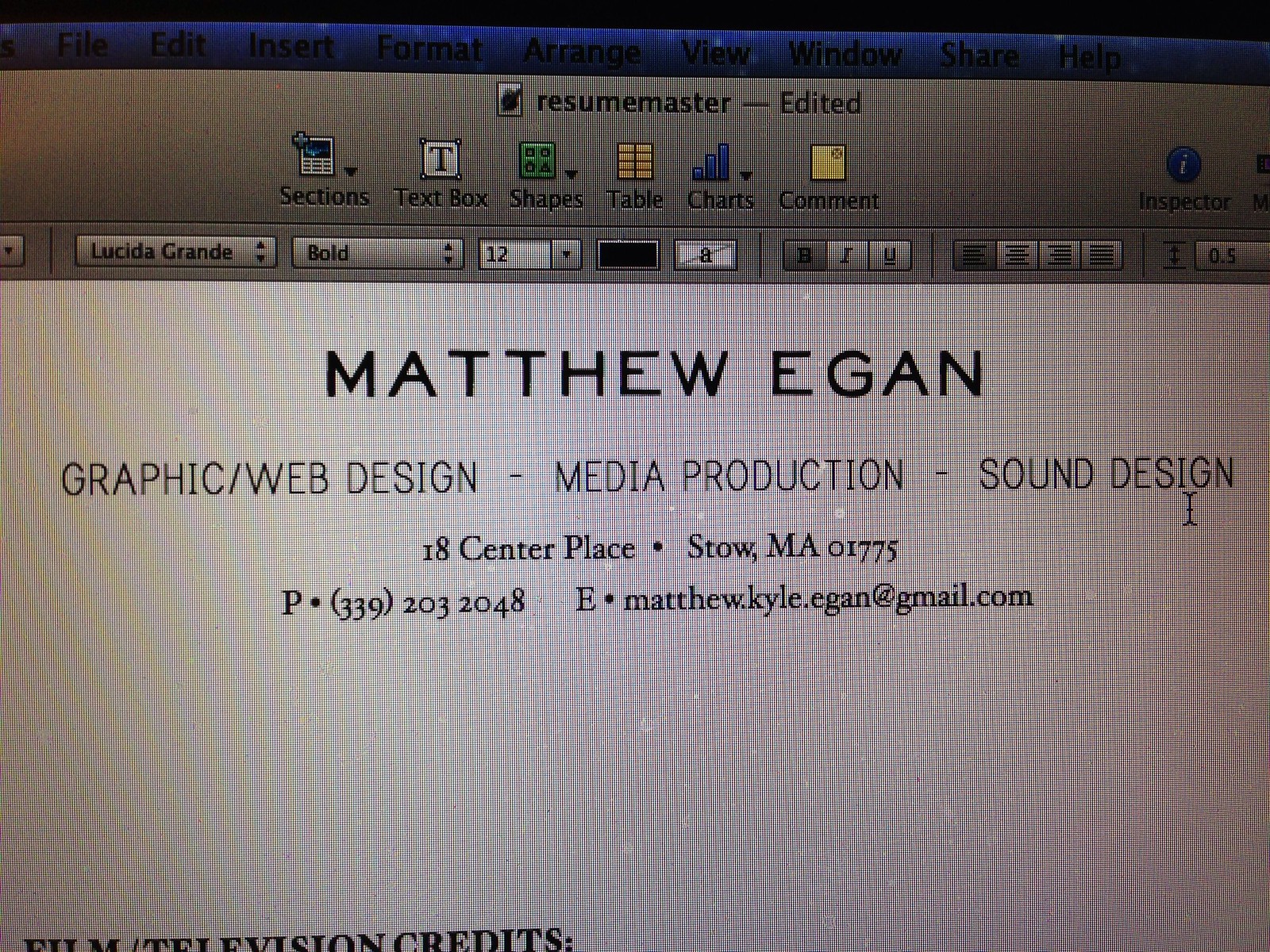The screenshot showcases a computer screen displaying a software interface titled "Resume Master - Edited." At the top, there is a blue horizontal strip with tabs labeled File, Edit, Insert, Format, Arrange, View, Window, Share, and Help. Below this strip, in a gray section, it says "Resume Master - Edited," followed by icons for Sections, Text Box, Shapes, Table, Charts, Comments, and Inspector. This area is accompanied by formatting tools, including font options like Lucida Grande, font size, bold, italic, underline, and alignment buttons. The main white area of the screen prominently displays the name "MATTHEW EGAN" in all caps, with details beneath listing Graphic/Web Design, Media Production, and Sound Design. The address is given as 18 Center Place, Stowe, MA 01775, with the phone number 339-203-2048, and email Matthew.Kyle.Egan@gmail.com. The lower left corner of the screen begins to show additional resume content, starting with "Film/Television Credits." The image is grainy, resembling a pattern of black and white small checks.